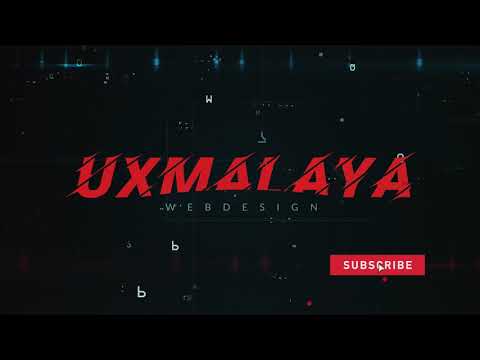The image features a somewhat futuristic and pixelated dark black background peppered with faint blue lights, resembling lens flares and refracting light. Floating within the space are small white letters—noticeably, two lowercase B's at the bottom and a W near the top. Dominating the center of the image is large red text that reads "UX Malaya," while directly below in smaller gray capital letters, it states "Web Design." In the bottom right corner, there is a prominent red rectangular button with white text that says "SUBSCRIBE." The overall composition gives it a modern and digital aesthetic, likely signifying a web design company.